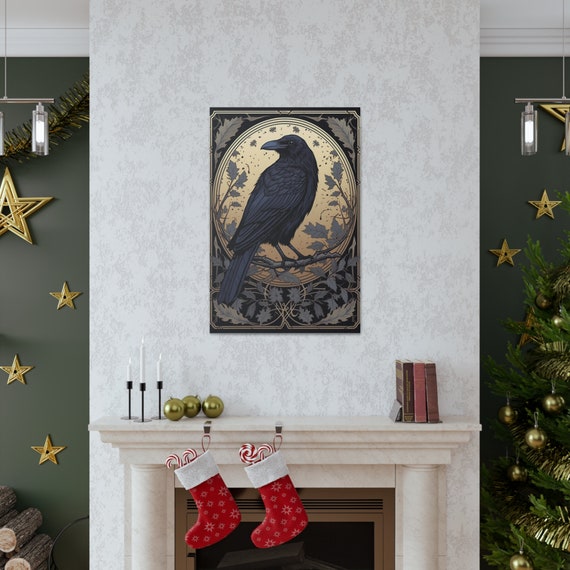This photograph captures a cozy, decorated fireplace scene against a textured wall. Central to the image is a striking graphic portrait of a raven on a golden background adorned with black and gold leaves, which hangs above the white mantle. The mantle is festively decorated, featuring three groupings of ball ornaments, three candles, and a small stack of books on the far right. Two red and white Christmas stockings, each holding a candy cane, dangle from the mantle. Below, logs are arranged on the left side, ready for a fire. Flanking the centerpiece are dark green walls embellished with golden stars, contrasting with the predominantly white and gray interior. To the far right, the edge of a Christmas tree with golden bulbs and decorations is visible, contributing to the holiday atmosphere.